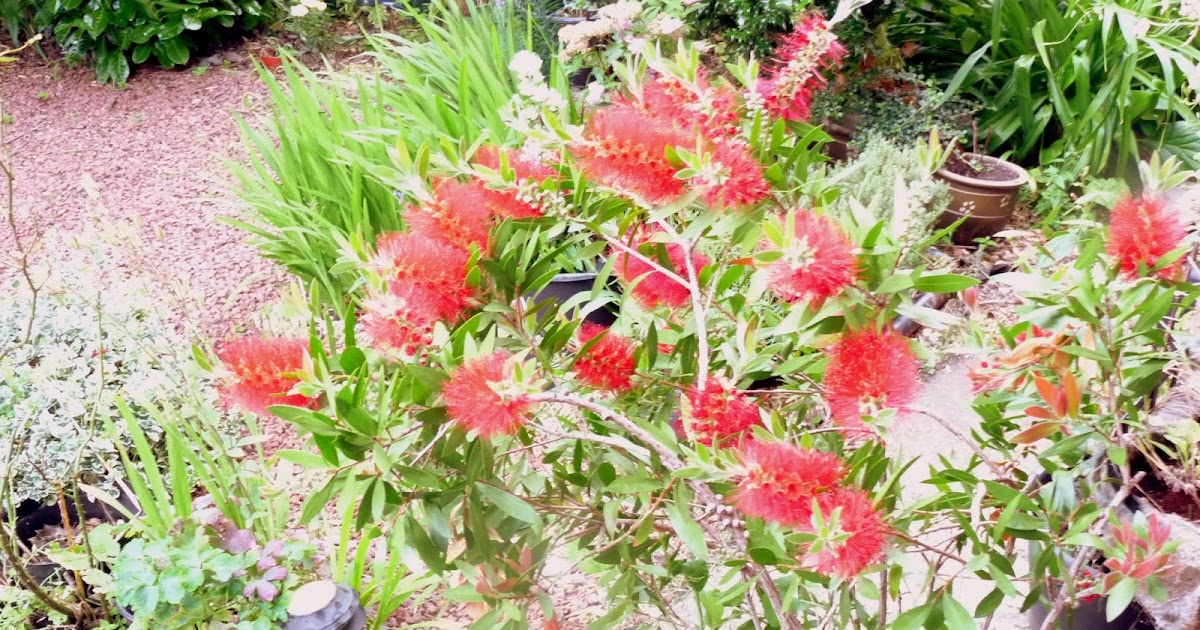The image depicts an outdoor garden scene rich with a variety of plant life. Central to the composition is a vibrant green plant crowned with pink and red flowers emerging from a mix of fuzzy sprigs, possibly identifiable as a butterfly bush or Monarda. The plant's woody stems stand prominently amidst lush greenery. Surrounding this focal point are various other plants, including shorter bushes close to the ground in the lower left, and narrow, lanky shoots in the upper right. The soil, a mix of red and brown hues, appears rich and possibly rocky, lending a slightly rugged texture to the garden pathway. Framing the scene in the background are darker green leaves of a shrub seen in the upper left, and a brown plant pot adorned with floral designs positioned in the back. The garden's abundant green foliage and diverse plant shapes create a picturesque and tranquil natural setting.